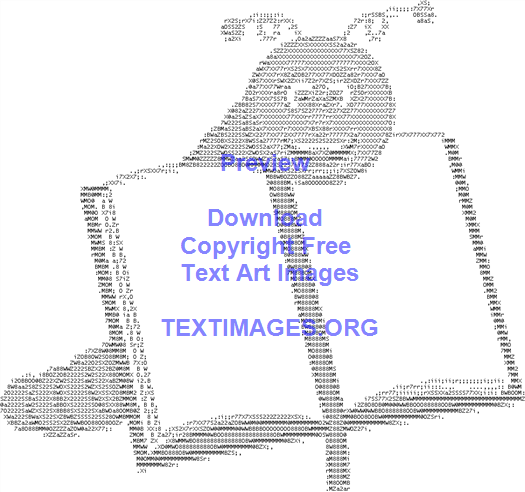The image depicts a cheerful caterpillar with a big smiling face, created entirely out of ASCII text—a style where various letters, numbers, and symbols are used to form a picture. The caterpillar has two antennae, two large eyes, and is made up of characters like question marks, number sevens, zeros, and twos. It is leaning over an upright book, resting its chin on the top edge of the book. The book features a bookmark draping down from the bottom and has a dark outline. In blue text above the caterpillar, the words "Preview, Download, Copyright-Free Text Art Images" are written, followed by a URL at the bottom that reads "textimages.org." The detailed and playful nature of the image gives it a whimsical, childlike appearance, reminiscent of illustrations found in children's books.